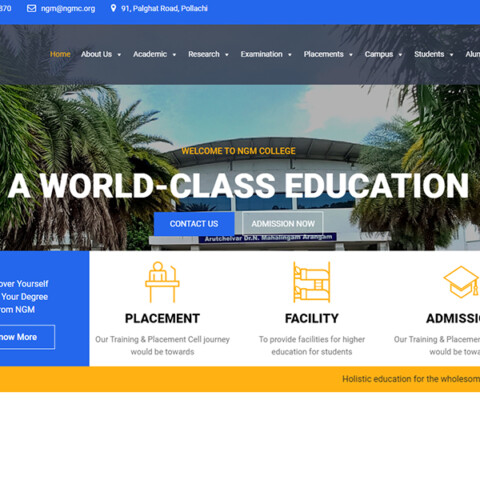This image showcases the homepage of NGM College's website, emphasizing its commitment to providing a world-class education. The backdrop features iconic palm trees flanking both sides, creating a serene and inviting atmosphere. Centrally positioned, a dome-shaped building prominently displays the welcoming message: "Welcome to NGM College." The website's navigation bar at the top includes tabs labeled Home, About Us, Academic Research, Examinations, Placements, Campus, and Students, facilitating easy access to various sections.

Highlighted at the top of the page is the college's address: 91 Palgett Road, Polachi, accompanied by a call-to-action box encouraging visitors to "Contact Us" for admissions. Below this section, three distinct icons offer additional information: a yellow figure seated at a table representing "Placement," a bunk bed icon indicating "Facility," and a graduation cap symbolizing "Admissions."